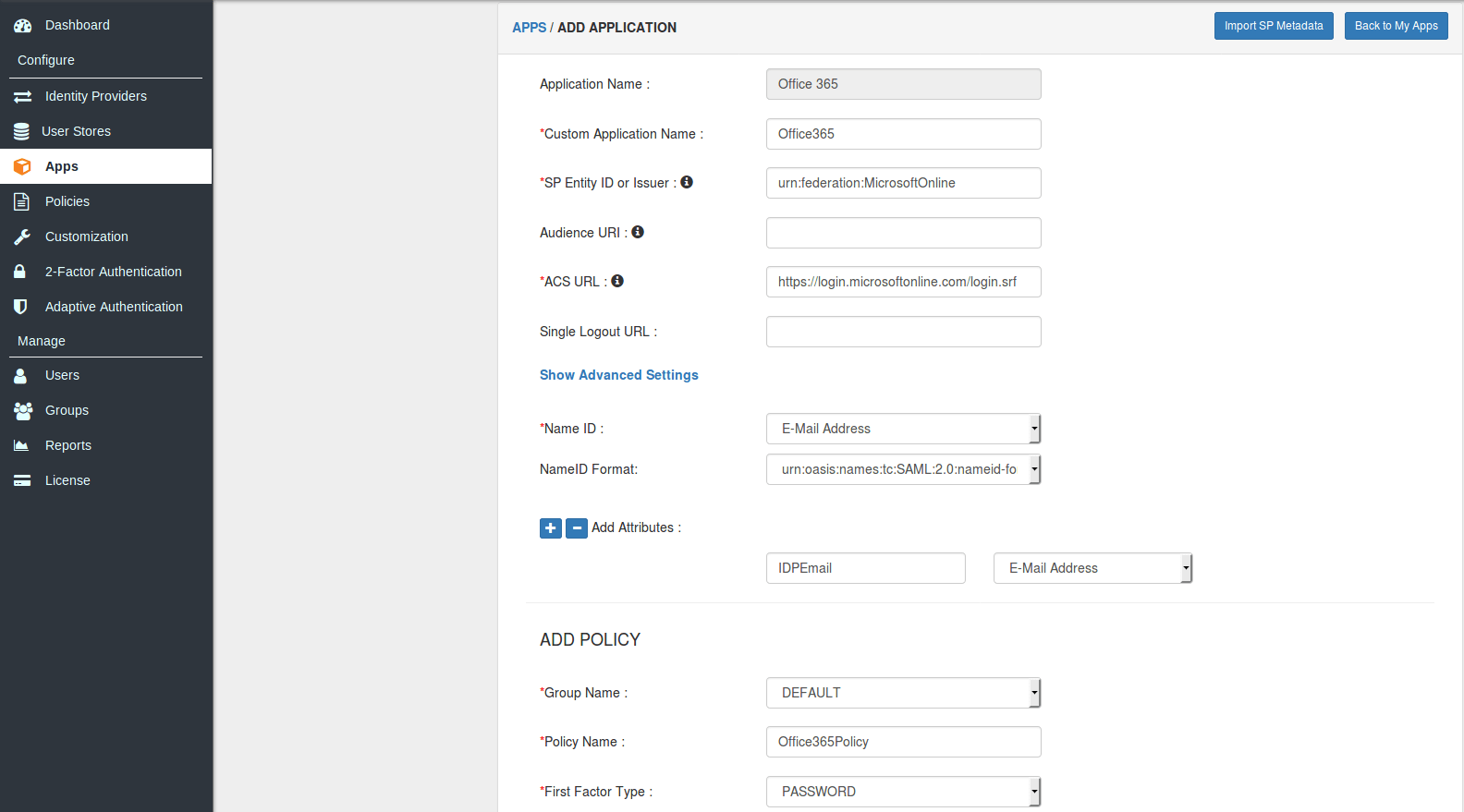A detailed view of a settings screen for a software application or website is presented. The layout is segmented with a dark steely blue vertical menu bar on the left, featuring white text for easy readability. The menu is divided into two main sections: "Configure" and "Manage". Each menu item is accompanied by an icon that visually represents its function.

At the top of the menu under "Configure," a dashboard icon resembling a speedometer leads to the Dashboard. Other options listed under "Configure" include Identity Providers, User Store, Apps, Policies, Customization, Two-factor Authentication, and Adaptive Authentication. The "Manage" section contains options for Users, Groups, Reports, and Licenses.

The main content area on the right side shows the details for adding an application. At the top, a header indicates the user is in the "Apps" section with a specific focus on "Add Application."

Two prominent blue buttons labeled "Import SP Metadata" and "Back to My Apps," both with white text, provide key actions. Below this, a form presents various fields, some pre-filled. These fields include Application Name, Custom Application Name, SP ID or Issuer, Audience URI, ACS URL, and Single Logout URL.

An option to "Show Advanced Settings" is available, revealing further customization options such as Name ID and Name Format. The form features various input methods including drop-down menus, text fields, and buttons.

For this particular instance, the application being added is Office 365. Additional configuration options include a section labeled "Add Policy," which requires input for Group Name, Policy Name, and First Factor Type, each accompanied by drop-down boxes and text fields to complete the setup.

Overall, the interface is detailed and structured to facilitate the setup and management of applications and their associated policies within the system.